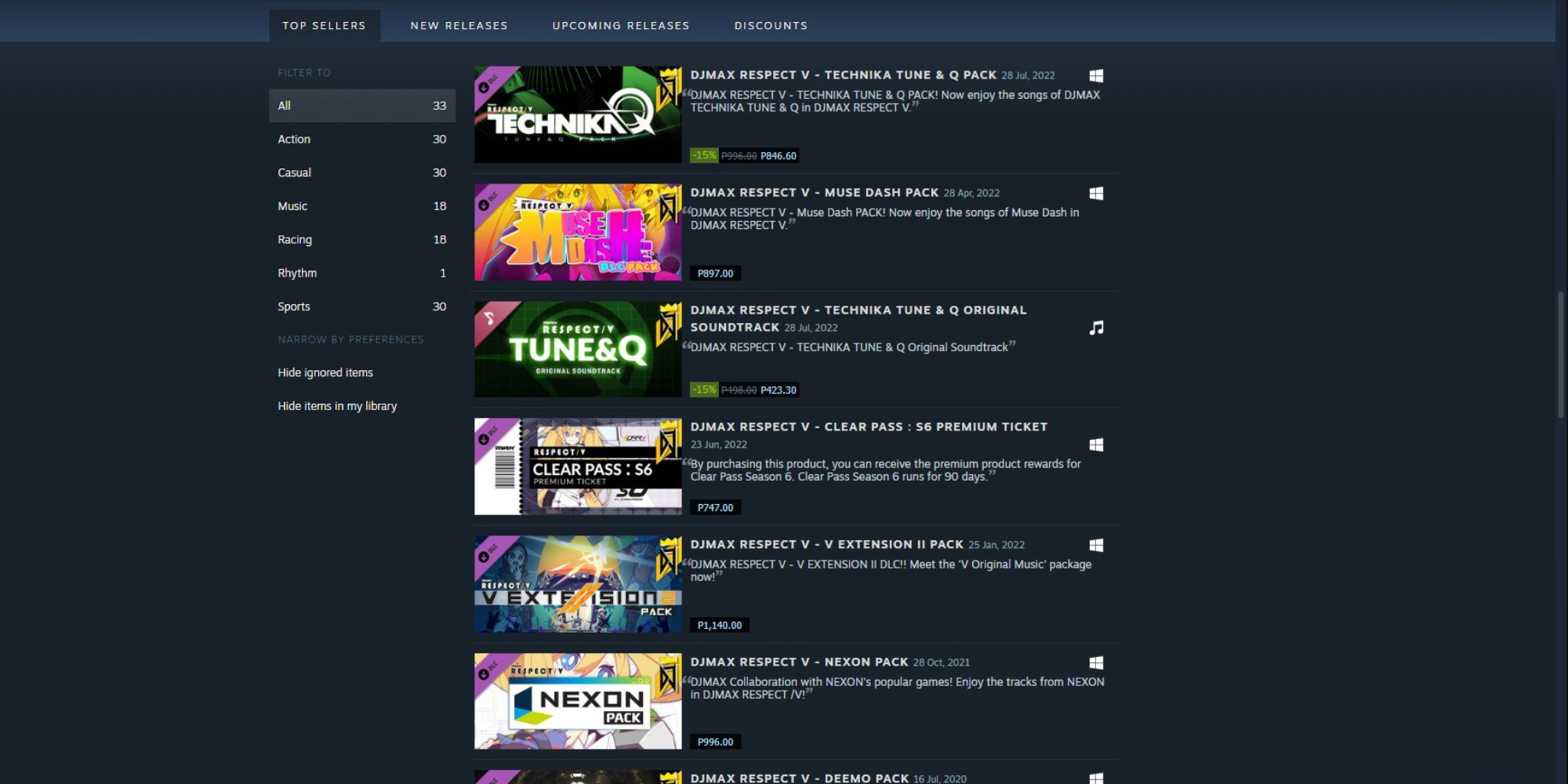This image displays a screenshot of a digital storefront, likely tailored for video games or software. At the top of the screen is a navigation menu with several categories: 'Top Sellers' (currently selected), 'New Releases,' 'Upcoming Releases,' and 'Discounts.' 

Below this menu, a series of tabs categorize the items, including 'All,' 'Action,' 'Casual,' 'Music,' 'Racing,' 'Rhythm,' and 'Sports.' The display is configured to 'Sort by Preferences,' with options to 'Hide Ignored Items' and 'Hide Items in My Library.'

The main section of the screen showcases several items, primarily related to the DJMAX Respect V series:

1. **DJMAX Respect V Technika Tune & QPAC**: Displayed with a distinctive Technika icon.
2. **DJMAX Respect V Muse Dash Pack**: Identified by a purple and yellow icon.
3. **DJMAX Respect V Technika Tune & QOriginal**: Marked with a green icon.
4. **DJMAX Respect V Clear Pass 56 Premium Ticket**: Accompanied by a black and white icon.
5. **DJMAX Respect V Extension II Pack**: Denoted by a blue and yellow icon.
6. **DJMAX Respect V Nexon Pack**: Noted with the text "Nexon" and an associated icon.

Each item in the list features its title and a corresponding unique icon, offering a clear visual representation for the user to browse through the available options in this digital store.